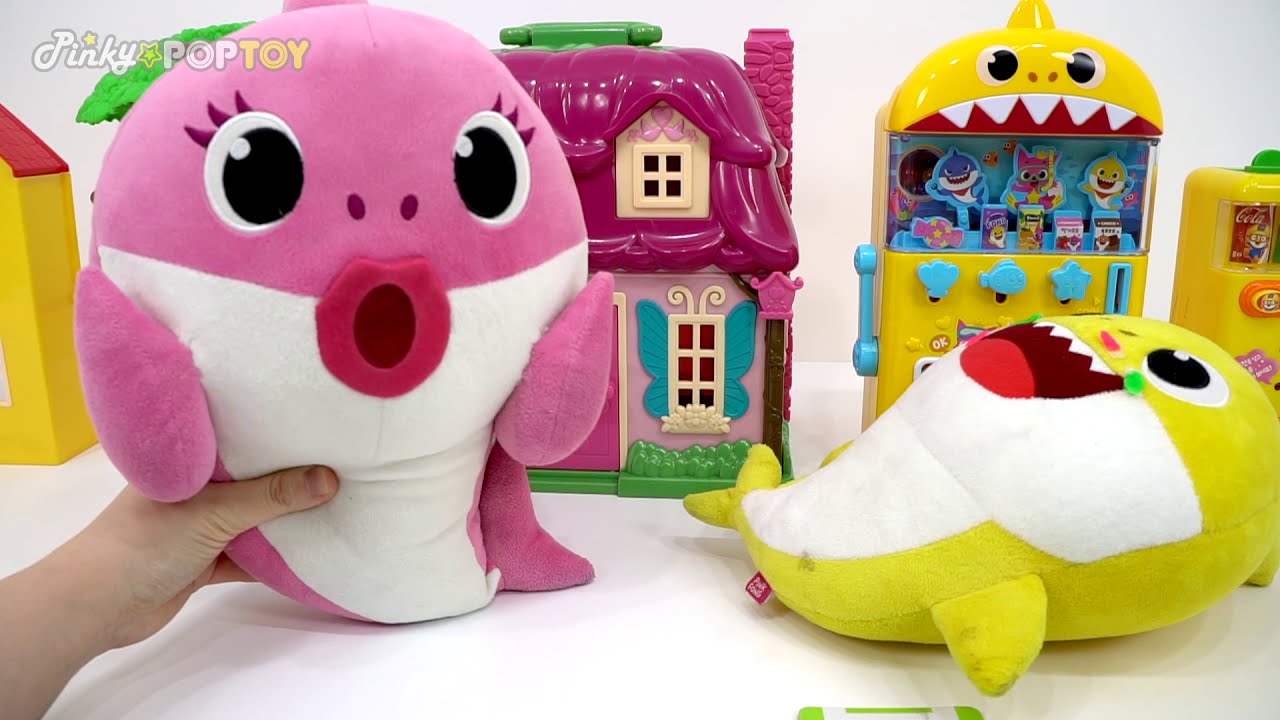This image depicts a series of colorful children's toys prominently labeled "Pinky Pop Toys" in a semi-transparent logo at the top left corner. Set against a stark white backdrop and a white tabletop, the scene is anchored by a hand entering from the left, delicately holding a plush toy that resembles a pink shark with a girl's face. This toy features a pink upper body with giant white eyes framed by three eyelashes on each eyelid, black pupils, and big red lips forming a round mouth. The pink plush has pink fins, a pink flipper, and a white underside. To its right, another plush toy lies on its back; this one resembles a yellow shark with similar large eyes, an open mouth displaying a red tongue and white teeth, and a white underbelly. Identifiable gender distinctions might suggest them as a girl and boy shark respectively.

Behind these two plush toys, there’s a collection of plastic accessories that complement the set. On the left, a pink plastic dollhouse with a green handle, detailed with window shutters and a bow atop the upstairs window, stands in view. Adjacent to the dollhouse, a yellow toy that appears like a shark's mouth, featuring a recessed section with blue and orange or yellow accents, buttons, and dowels, possibly functions as an engaging slot machine. All elements together create a lively and inviting playful scene, suggestive of an imaginative and interactive play set.